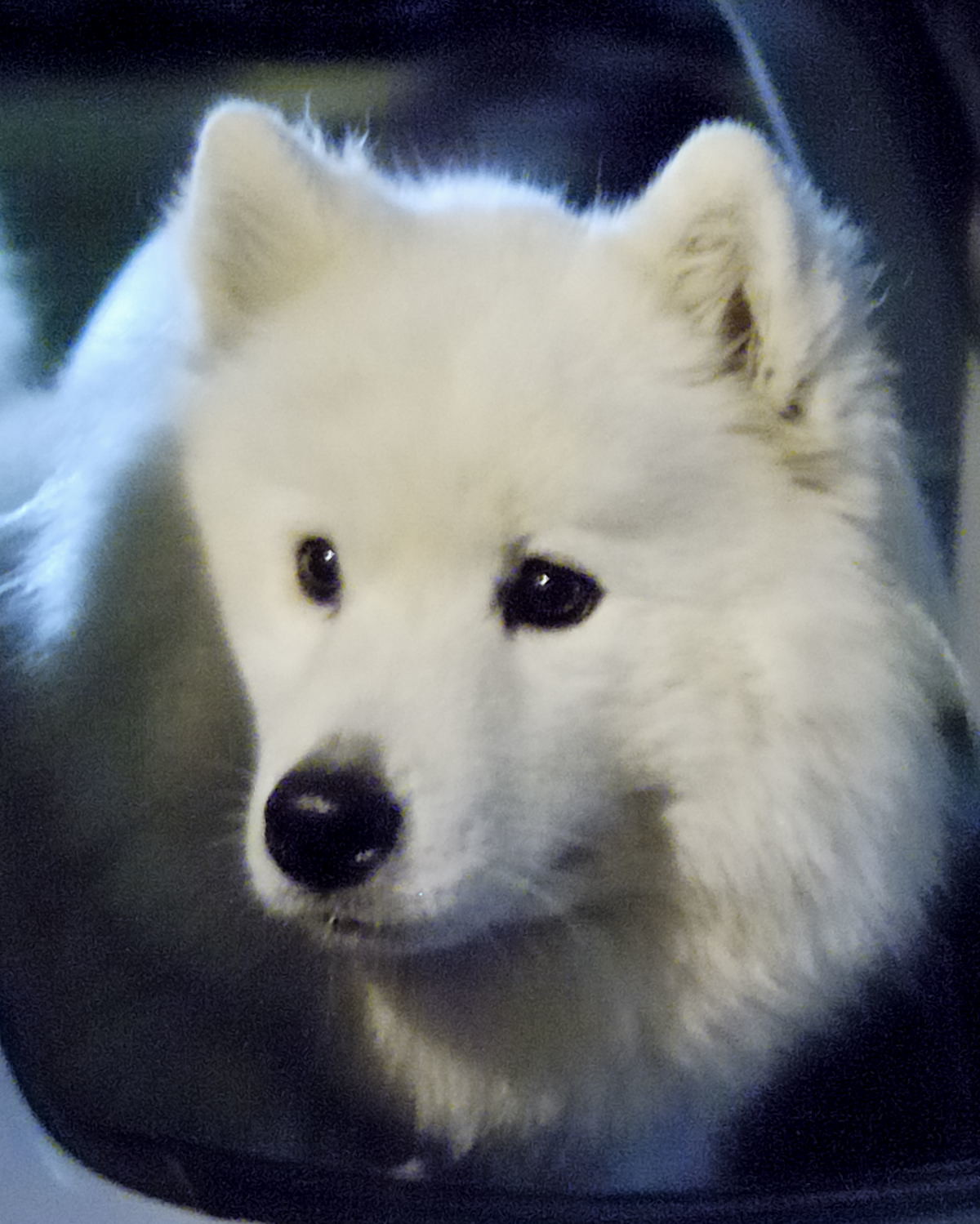The photo features a small, white, fluffy dog that looks like a puppy or a white husky mix with a general husky-shaped head. The dog has pointy ears, small dark eyes, a black nose, and fuzzy fur that poofs out on the sides. It's looking towards the bottom left corner of the image, seemingly staring off into the distance. The dog's ears stick out, and one ear reveals a small black spot inside. The dog appears to be sitting in a container of some kind, possibly in a vehicle, as evidenced by the black outline and rubber-like material visible at the bottom of the image. A white chunk in the bottom left corner further suggests it might be inside a car. A slight shade falls on the dog from the object containing it, adding depth to the scene.